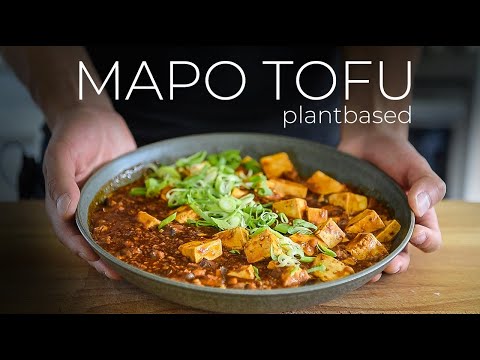This horizontal, color photograph features a dark, advertisement-like aesthetic with a black background and a narrow black stripe running across the top and bottom. Dominating the center of the image is a bluish-gray plate, held by two hands wearing a black shirt, which are in the process of setting the plate down on a wooden table. The plate, which could be described as bowl-like, contains an appetizing display of cubes of white tofu nestled in a rich red sauce. Green scallions are visibly arranged down the middle of the dish, adding a splash of color and contrast. Above this mouthwatering scene, white letters prominently announce "Mapo Tofu," followed by the descriptor "plant-based," emphasizing the dish's vegan attributes.